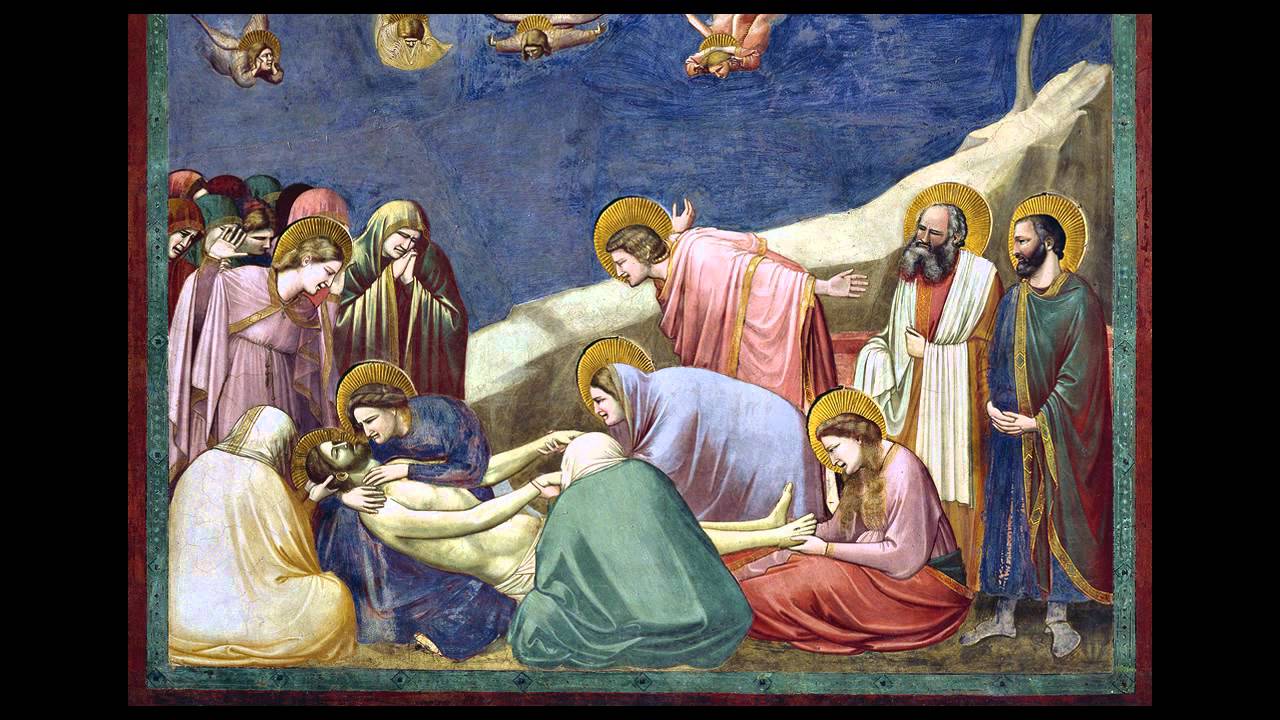The painting vividly portrays the solemn scene of Christ being taken down from the cross, an iconic moment fraught with both sorrow and reverence. At the center, Jesus, identifiable by his brown beard and long hair, is cradled by a woman in a blue dress, likely the Virgin Mary, who tenderly supports his torso, her face close to his. Surrounding her are several distressed women, one clutching his feet, another holding his hands, while another embraces his neck. Two of Christ's disciples stand to the right side, helping prepare him for burial. High above, a choir of four angels with bird-like wings hovers in a serene blue sky, underscoring the divine nature of the scene. Many figures, including Jesus and his immediate mourners, are depicted with golden halos, symbolizing their sanctity, while a group of concerned onlookers without halos gathers on the left, reflecting the universal grief and doubt surrounding this poignant moment. The painting's rich color palette includes not only predominant blues and whites but also touches of green, purple, pink, gold, and orange, enhancing the emotional depth and sacred atmosphere of the artwork.